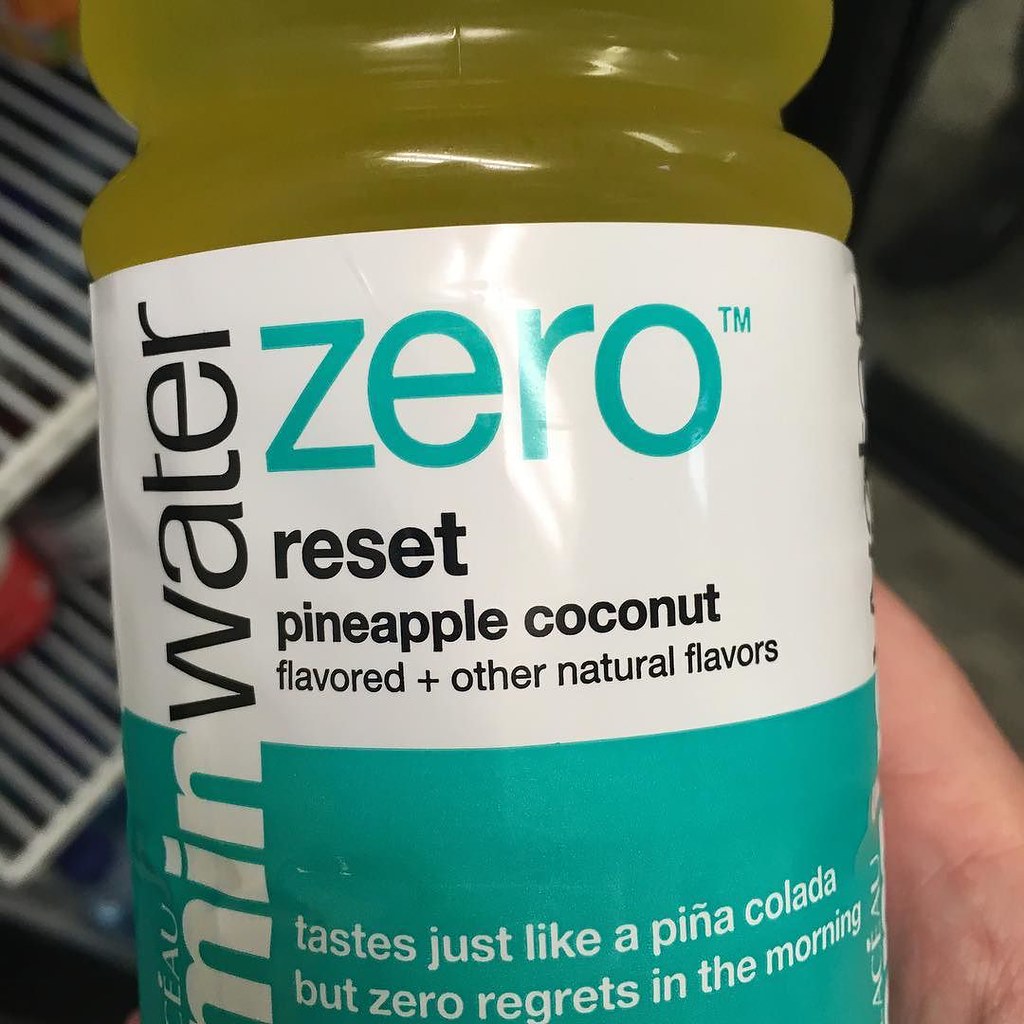The image features the interior shelves of a refrigerator, identifiable by the metallic, hole-covered vents in the background. A dark-colored floor is visible below. In the foreground, a person's hand is holding a plastic bottle. The bottle sports a white label with a greenish-blue lower section. In black text on the white area of the label, it reads "Men Water" and "Zero." Beneath this, it states "Reset Pineapple Coconut Flavored plus other natural flavors." On the greenish-blue portion of the label, white writing claims, "Tastes just like a piña colada but zero regrets in the morning." A small red object can also be seen on one of the refrigerator shelves.